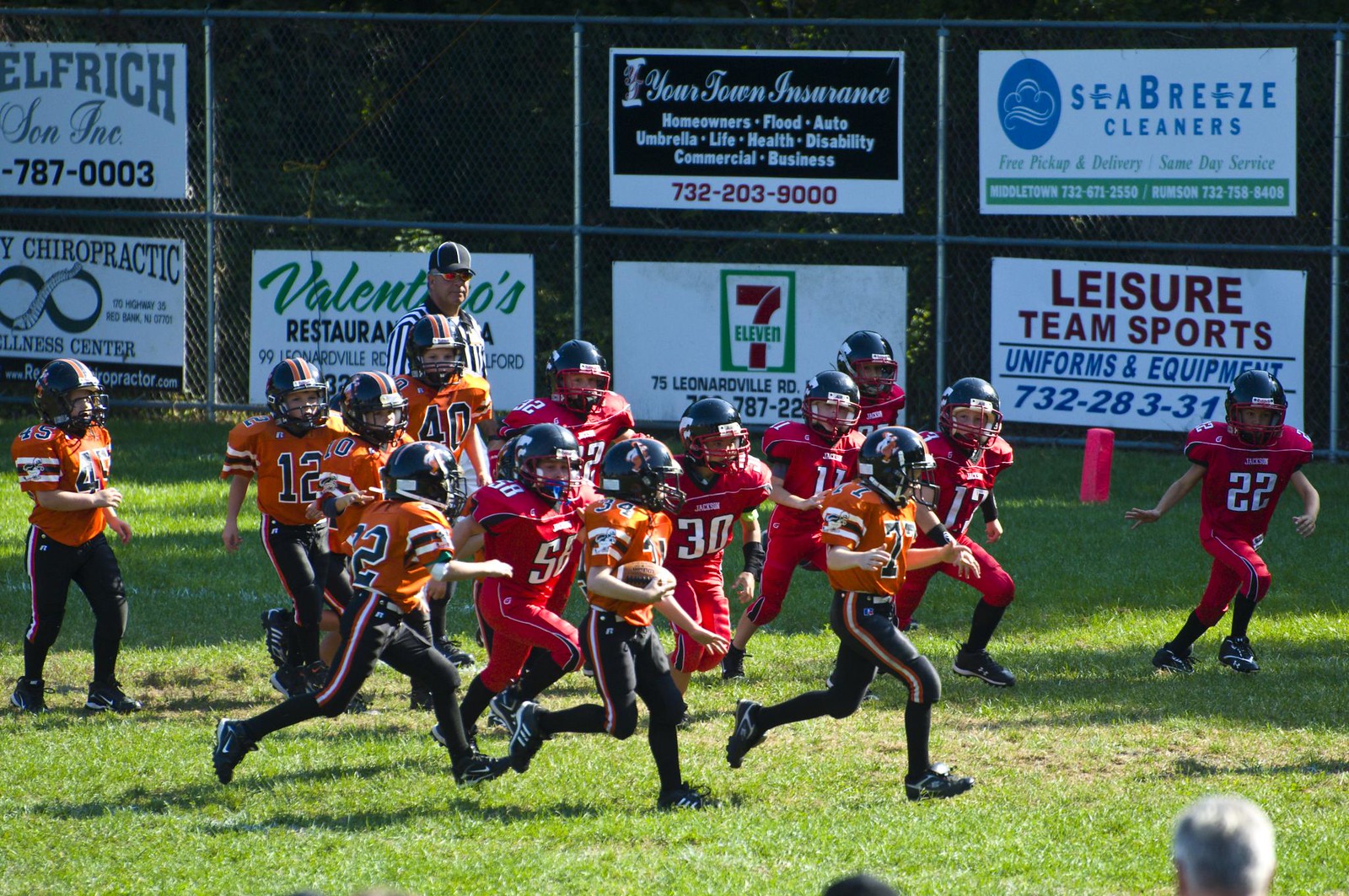The image captures a dynamic moment in a youth football game under a sunny sky. On a vivid green field, two teams—one in orange jerseys with black pants and the other in red jerseys—are fully engaged. Both teams don black helmets. A player from the orange team is sprinting with the football cradled in their right arm, heading towards the end zone marked by a red pylon. Trailing closely behind, players from the red team are in hot pursuit. On the left side of the image, a referee stands watch in uniform, while a chain-link fence in the background displays various advertising billboards, including ones for "Sea Breeze Cleaners," "Leisure Team Sports," "7-Eleven," "Valentino's Restaurant," and a chiropractic office. Additional details include the heads of a gray-haired adult and a child peeking above the fence and distinct shadows on the well-maintained pitch, highlighting the sunny conditions.